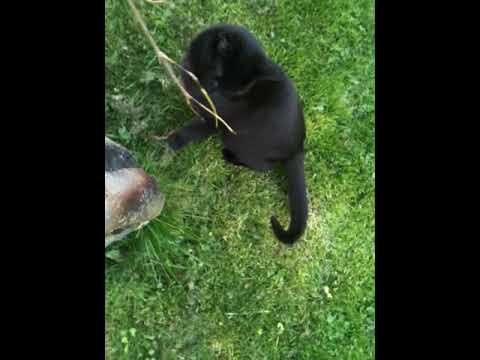This image captures a black cat with long fur, positioned at the very bottom edge of the frame, scratching its front paws on a tree stump or possibly a telephone pole. The stump has a very weathered, cylindrical appearance, extending vertically out of the top edge of the image. The cat is looking upward as it scratches, and its pose suggests a potential intention to climb. The photograph is taken at a shallow angle towards the ground, with the entire scene framed in a vertical cell phone style but rotated within a landscape-oriented format, resulting in black bars on the left and right sides. The setting appears to be a grassy area, possibly someone's backyard, complete with mulch and landscaping around the periphery, hinting at a fence visible at the upper right edge of the frame.